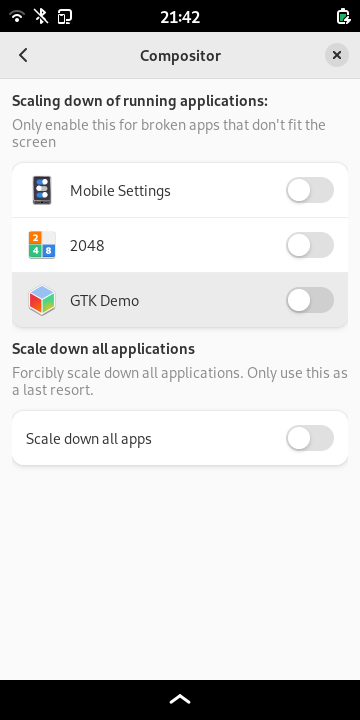This screenshot displays a settings page dedicated to application scaling within a compositor. The interface features a dark gray header bar labeled "Compositor," with a back arrow icon on the left and a close icon (X) encased within a gray circle on the right.

Directly below the header is a section titled "Scaling Down of Running Applications," written in bold. A subtext in light gray advises that this setting should only be enabled for applications that don't fit the screen. The main content area presents a list of three applications—Mobile Settings, 2048, and GTK Demo—each accompanied by a toggle switch that is currently set to off (indicated by gray).

Further down, there is an option labeled "Scale Down All Applications," followed by a warning text in light gray stating, "Forcibly scale down all applications. Only use this as a last resort." This is accompanied by a toggle switch labeled "Scale Down All Apps."

The background of the settings page is light gray, providing a neutral canvas for the various controls and texts. At the bottom of the screen, a black bar spans the width, featuring a white up arrow icon centered within it.